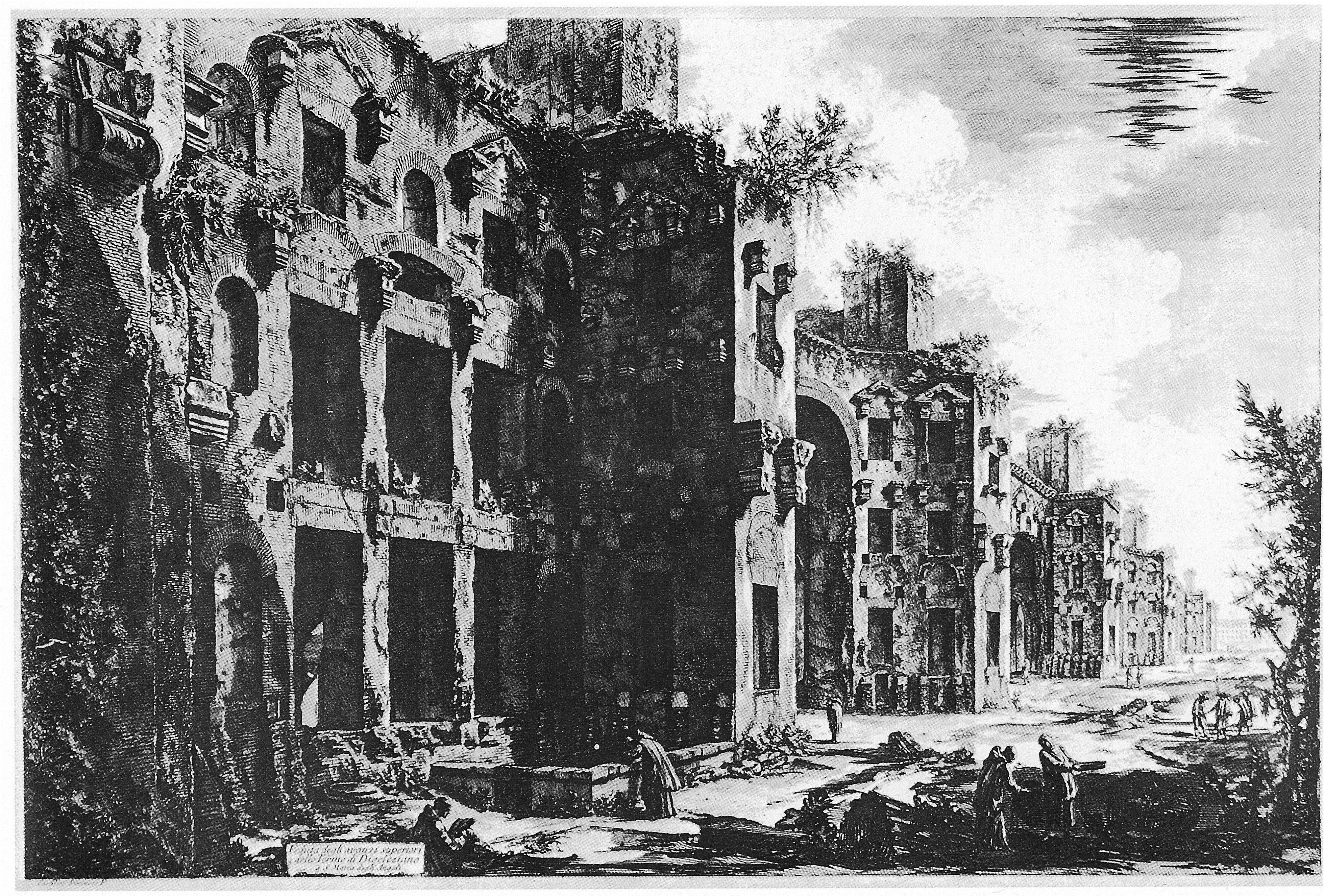The image depicts a black and white drawing of an old, possibly abandoned, three-story townscape. Dominated by large, ancient buildings with arch-shaped tops, the largest building on the left side features multiple huge windows and a central column-like structure too large for a chimney. This central structure might have historical significance or be part of the architectural design. Depictions of small, shadowy figures are scattered around, hinting at human presence. Notably, in the bottom right corner, there's a tree and clusters of people, suggesting some activity or gathering. The overall scene is set against a gray and white sky, partially obscured by black splotches which might represent a flock of birds in V formation or abstract artistic elements. Additional details include ivy scaling up the sides of buildings, suggesting the buildings have been in disrepair, and some indecipherable text at the bottom left, possibly attributing the artwork.